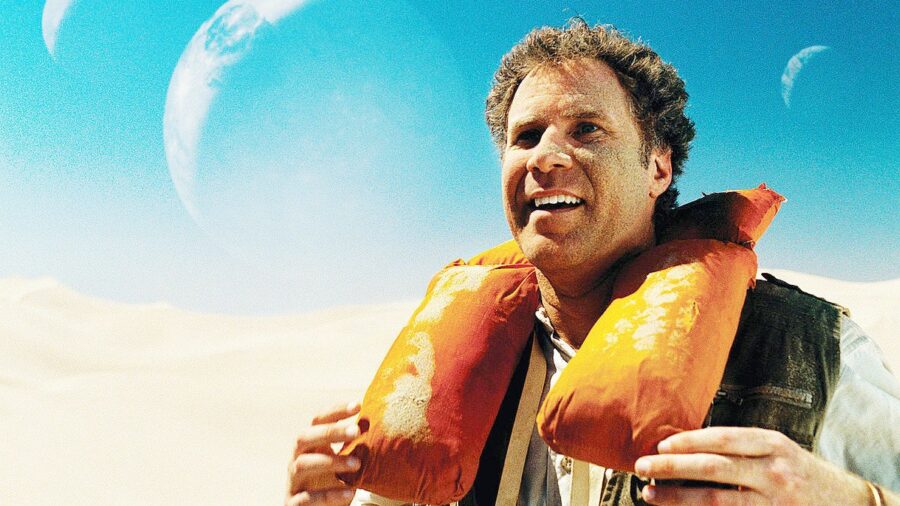In the image, we see Will Ferrell prominently positioned on the right side, wearing an orange life preserver around his neck. His life preserver is divided into two sections that rest on either side of his chest. Ferrell's hands grip the edges of the life preserver in front of him. He has medium-length brown hair with hints of gray and is sporting a light-colored shirt with gray vertical stripes, partially covered by a green vest. His expression is a casual smile as he faces slightly towards the left. The background features a series of small sand dunes under a bright blue sky. The sky is populated with three celestial bodies: a large planet on the center left, a smaller one to its left, and another moon or planet in the upper right. The image, which appears to be a film still possibly from the movie "Land of the Lost," exhibits noticeable film grain, particularly evident in the sky.